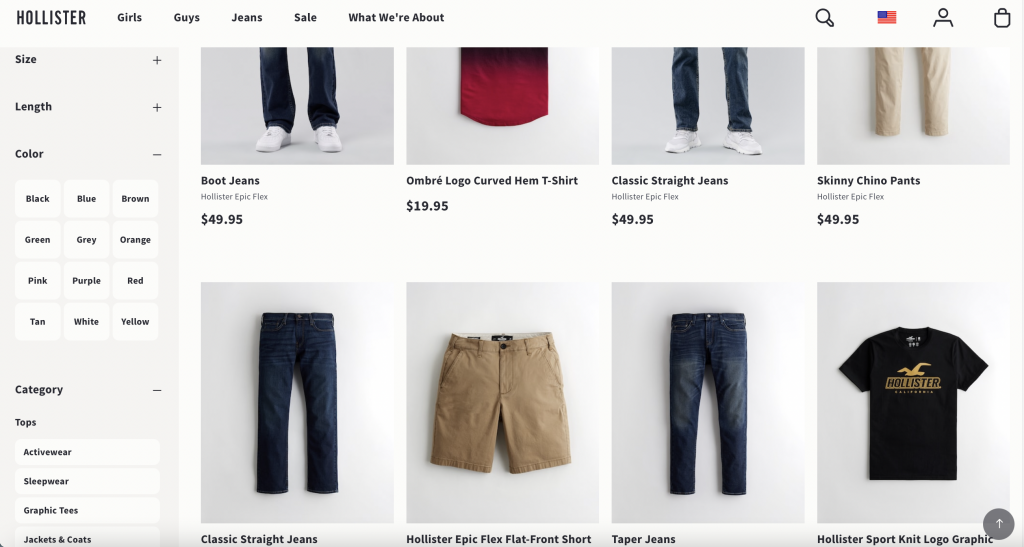This screenshot captures the web page of Hollister, an apparel company. At the top of the page, the brand name "Hollister" is prominently displayed. To the right of the brand name are navigation categories: "Girls," "Guys," "Jeans," "Sale," and "What We're About." Further to the right, there is a row of icons including a search icon, an American flag icon, a person/account icon, and a shopping bag icon.

On the left side of the webpage, there is a detailed filter menu. The menu allows users to narrow down their search by size, length, color, category, and specific types of clothing such as tops. Under the tops category, subheadings include activewear, sleepwear, graphic tees, jackets, and coats.

In the main section of the webpage, products are showcased in two rows of images. 

**First Row:**
1. Boot Jeans - $49.95
2. Ombre Logo Curved Hem T-Shirt - $19.95
3. Classic Straight Jeans - $49.95
4. Skinny Chino Pants - $49.95

**Second Row:**
1. Straight Classic Jeans (pictured with an image of jeans)
2. Hollister Epic Flex Flat Front Shorts (pictured with tan shorts)
3. Tapered Jeans (pictured with blue jeans)
4. Hollister Sport Knit Logo Graphic (pictured with a black t-shirt)

Each product listing includes both an image and the item’s name alongside its price, ensuring shoppers have a clear idea of what they are viewing and its cost.